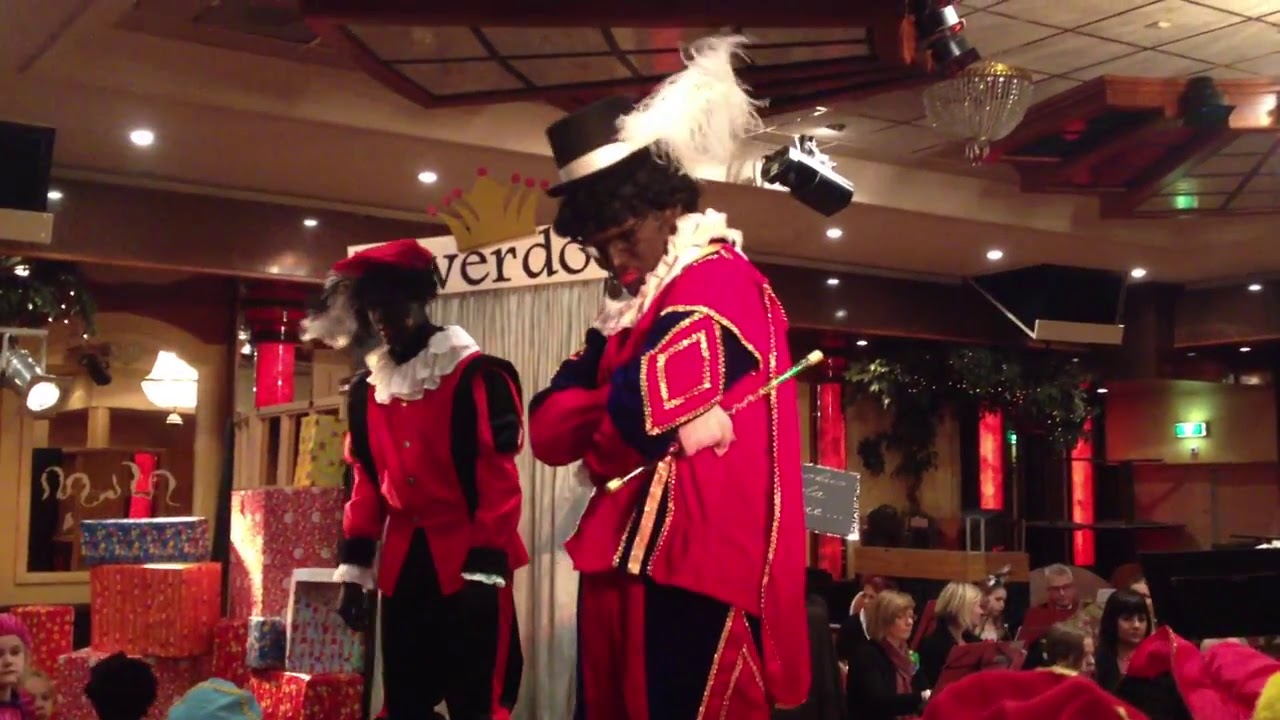In an indoor event hall adorned with stage spotlights and a white ceiling, two black gentlemen stand at the focal point, dressed in elaborate jester-like court costumes. Both wear ruffled cream-colored collars and distinctive hats adorned with feathers and ribbons. The central figure, slightly larger, dons a black top hat with a white feather and is dressed predominantly in red, featuring black-edged red diamonds at the elbows. He crosses his arms over his chest and holds a conductor's rod in his right hand, accentuating his theatrical stance. His companion to the left wears a red cap, with similar red and black attire but carries all-black pants. Behind them to the bottom right, a group of people is seated, potentially watching a performance. To the left, an array of cubical and rectangular prism-shaped wrapped presents lies scattered above which two small heads peek out, one in a pink hat. A banner with partially obscured text hangs above white curtains, completing the festive, theatrical atmosphere.